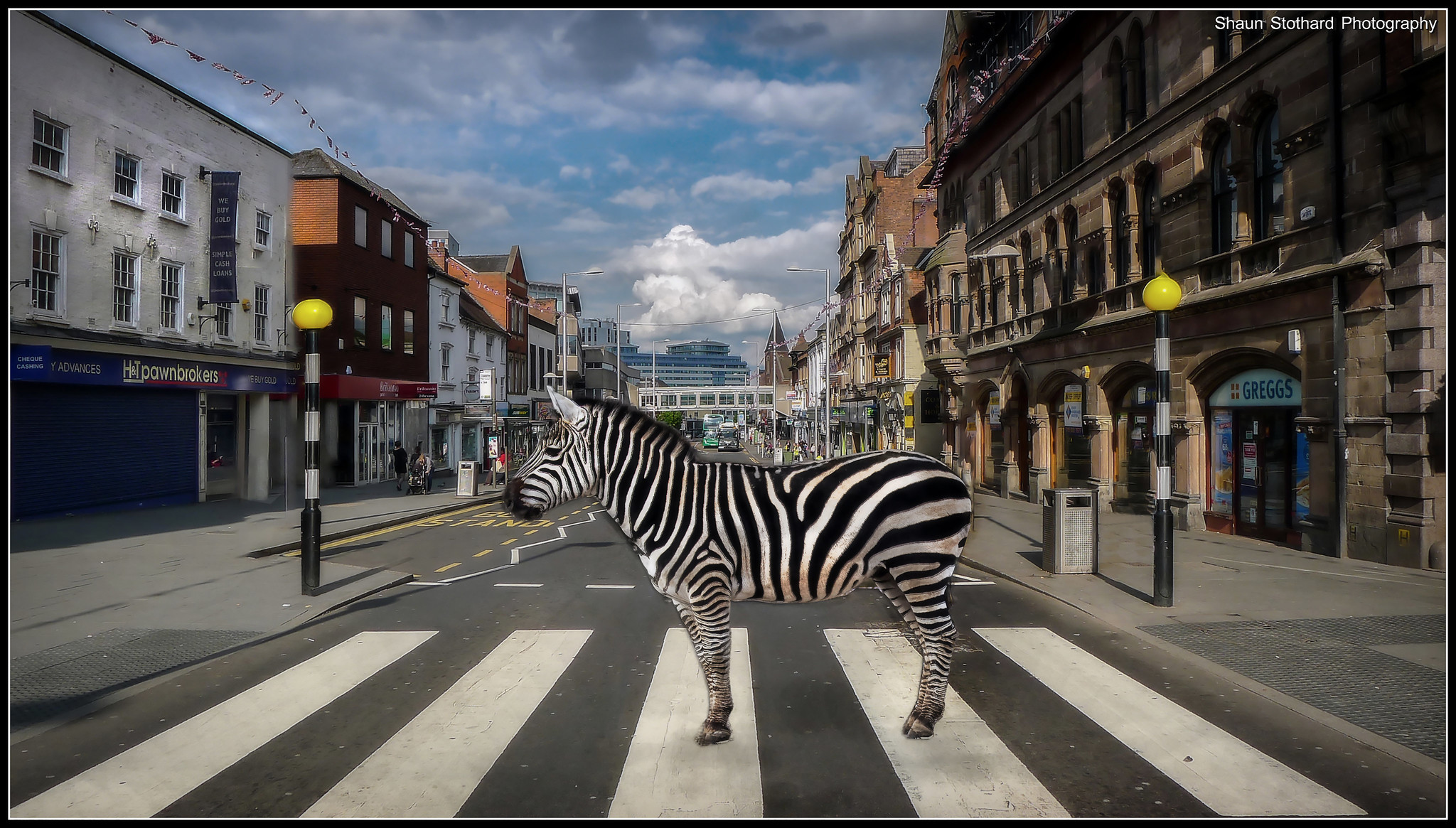This highly detailed photographic image captures a surreal scene set in a city or town street during the day. At the center of the composition, a zebra with striking black and white stripes stands on what appears to be a crosswalk, facing left. The street is notably deserted, devoid of any bustling traffic, lending an almost eerie quiet to the setting. On either side of the zebra, there are black poles with white stripes and round yellow globes at the tops.

To the left, the streetscape is lined with a series of low-rise buildings, predominantly three stories high, featuring various storefronts. The first building is white, with a sign partially visible that reads "PAWN." Adjacent to it is a brown building with wooden siding and a black roof. Further down the block, another white building and several white structures can be seen interspersed with red brick sections and red awnings. One notable structure has a brown gabled roof and there's another gabled roof to the left.

On the right side of the street, the architecture shifts to more stone-based structures. Prominently visible is a brownstone building with the sign "Greggs" spelled out in capital letters, accompanied by four red squares to the left of the text. Further down, the background reveals a series of stone buildings culminating in what appears to be a modern, bluish-grey structure. Beyond the buildings, two buses are seen approaching, with a silver subway car traversing a bridge above them.

The sky is a mixture of gray overcast clouds and patches of blue, offering a contrast to the otherwise muted cityscape. A watermark at the top right corner reads "Sean Stotthart Photography," adding an element of authenticity to the otherwise dreamlike composition. Notably, in the distance, a multi-story building and the steeple of what resembles a church or tower with a gabled roof punctuate the skyline. Despite the presence of typical city elements like buses and signage, the absence of people and cars near the zebra adds an abstract, almost animated feel to the image, making it both intriguing and surreal.